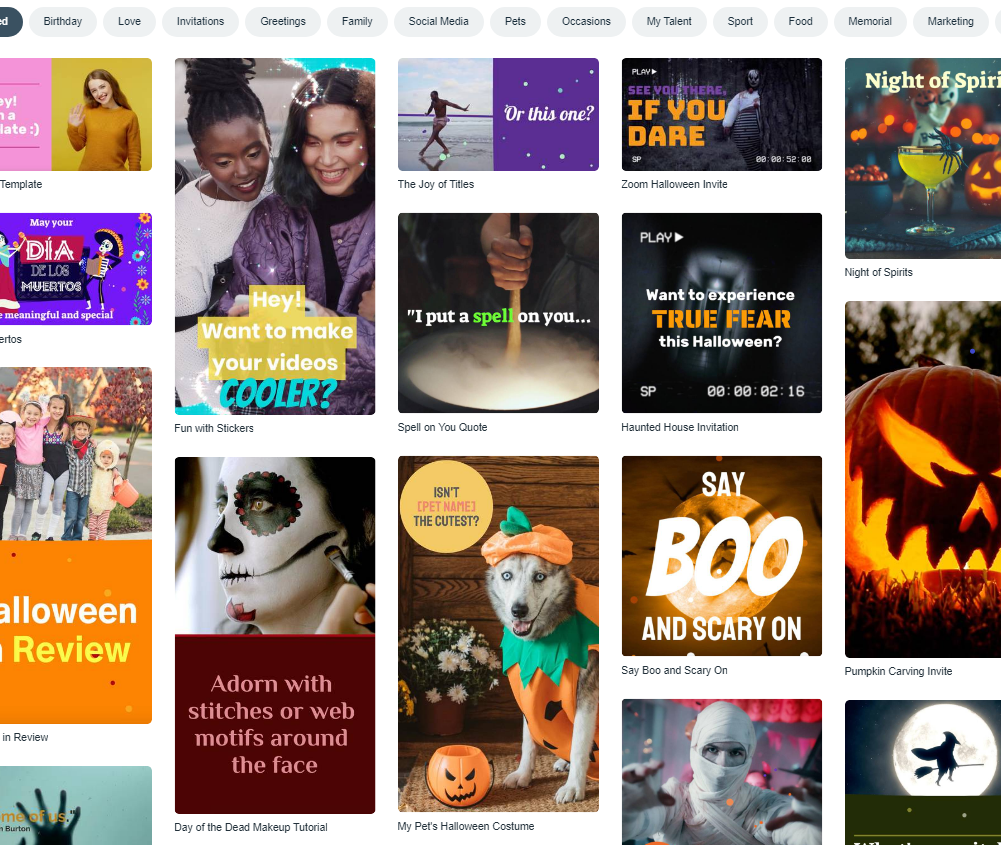The image displays a vibrant website interface with an array of headings sprawling across the top. Categories like Birthday, Love, Invitations, Greetings, Family, Social Media, Pets, Occasions, My Talent, Sport, Food, Memorial, Marketing, and others are clearly delineated. The selected category is on the far left, though partially obscured, it is evidently Halloween-themed due to the nature of the content displayed below.

Beneath these headings, a series of eye-catching, tile photographs are showcased, each evoking the essence of Halloween. The tile images include:
- A dog adorably dressed in a Halloween costume, labeled "My Pet’s Halloween Costume".
- A menacing ghoul draped in ragged attire.
- An image with the text "Say Boo and Scary On".
- A close-up shot of a pumpkin illuminated from within, captioned "Pumpkin Carving Invite".
- A mystical witch soaring past a glowing moon.

Each tile features a succinct description, enhancing the thematic coherence and guiding the viewer through the Halloween-centric digital display.